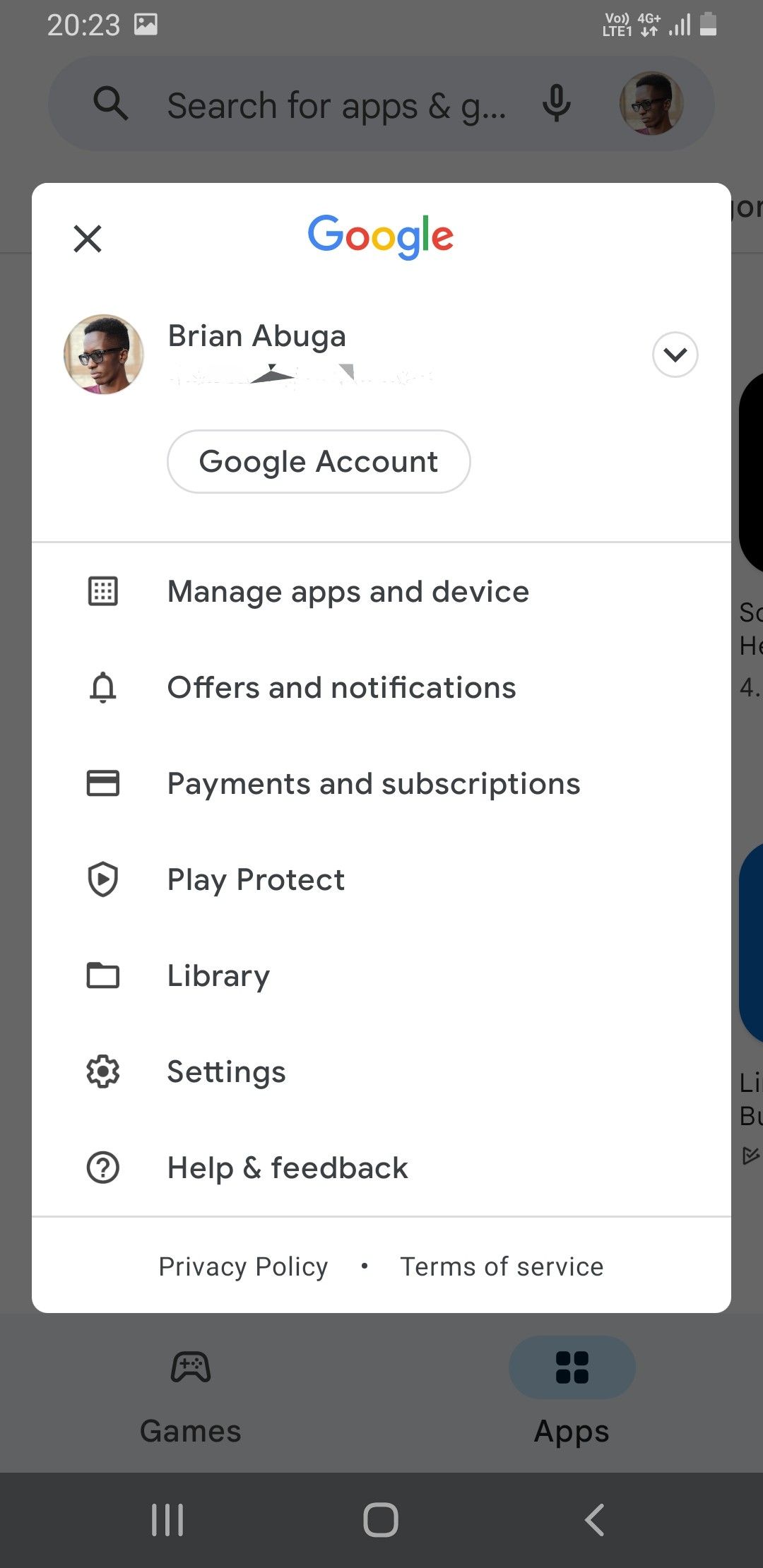Screenshot of the Google Profile Menu Interface

This screenshot captures the Google profile menu, prominently featuring a white overlay that occupies most of the webpage. At the top center, the Google logo is clearly visible, while an 'X' button for closing the menu is located in the top left corner.

Central to the overlay is the profile section, where the name "Brian Abuga" is displayed. Positioned to the left of the name is a circular profile picture depicting a black male with short hair and glasses. Adjacent to the profile picture, on the right, is a drop-down menu indicated by a down arrow.

Beneath the profile section, there is a pill-shaped button labeled "Google Account." Following this, a horizontal line demarcates the separation from the subsequent list of options, which include:

1. Manage Apps and Devices
2. Offers and Notifications
3. Payments and Subscriptions
4. Play Protect
5. Library
6. Settings
7. Help and Feedback

At the bottom of the menu, links to the Privacy Policy and Terms of Service are provided.